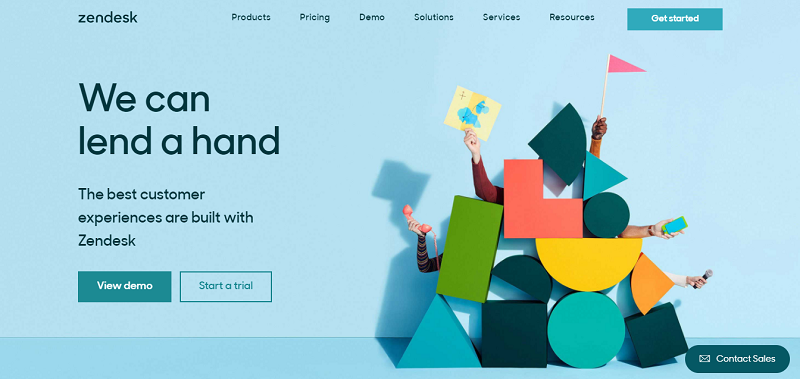The screenshot depicts a section of a computer screen with a light blue background, prominently featuring the Zendesk homepage. In the upper left corner, the logo "Zendesk" is displayed, followed by a navigation bar that stretches to the right, listing options for Products, Pricing, Demo, Solutions, Services, and Resources. Adjacent to these options, a prominent teal button labeled "Get Started" is situated.

On the left-hand side of the screen, a headline in bold text reads, "We can lend a hand, the best customer experiences are built with Zendesk." Below this headline are two call-to-action buttons: one on the left in a darker blue hue labeled "View Demo," and another on the right in a lighter blue shade that says "Start a Trial."

The right side of the screen is adorned with an artistic arrangement of geometric shapes, including a green rectangle, a yellow semicircle, a blue circle, a blue triangle, and a square. Emerging from behind these shapes are several hands and arms: two on the left, one at the top gripping a pink flag, and two more on the right, adding a touch of human interaction to the scene.

In the bottom right corner, a dark blue oval button features an email icon, accompanied by the text "Contact Sales" in white lettering.